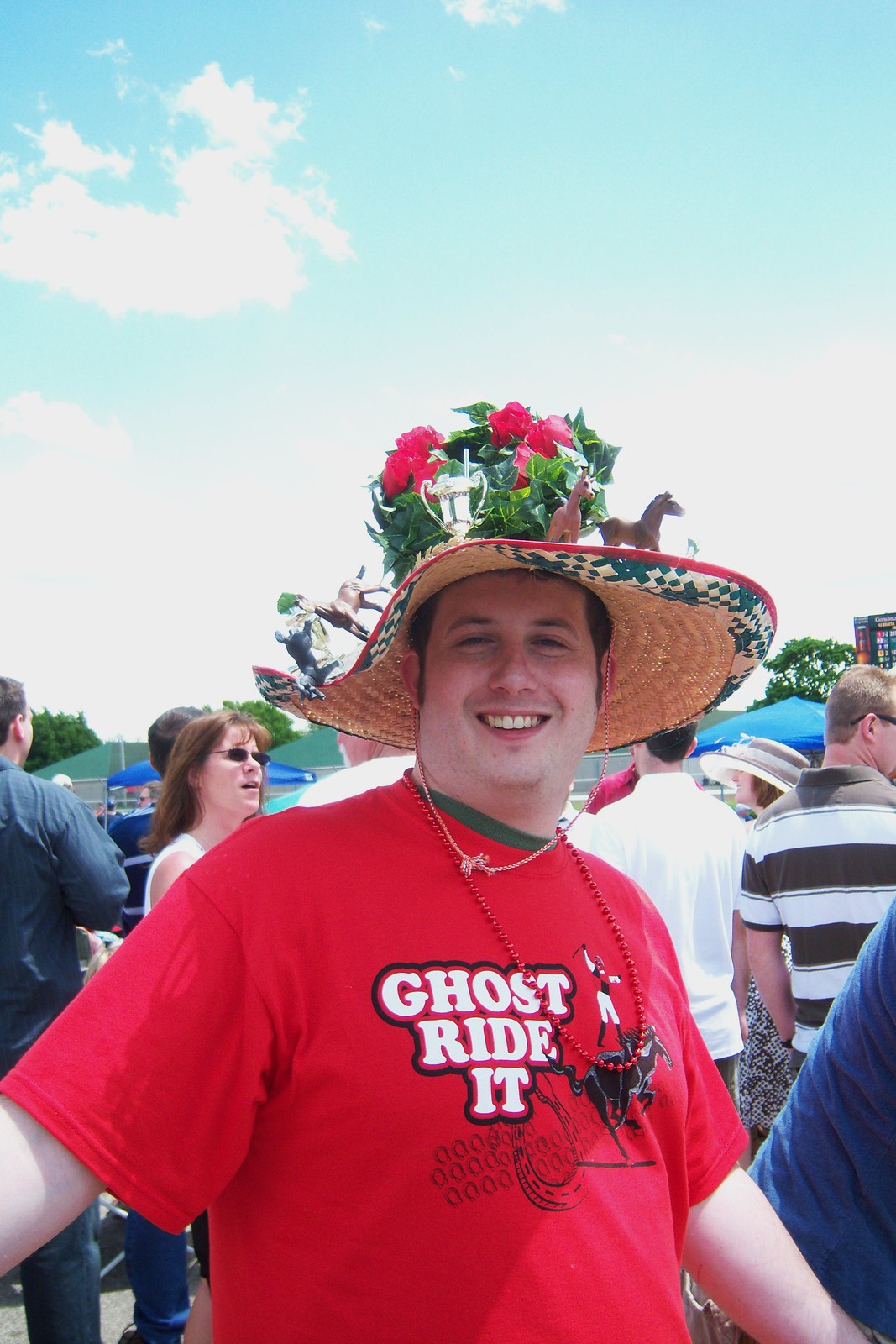In this vibrant image, a young, smiling Caucasian man is seen standing outdoors from the waist up. He is dressed in a bright red short-sleeved t-shirt featuring a design of a person standing on the back of a horse with their arms raised, accompanied by the text "Ghost Ride It" on the left. Adorning his neck are red beads, adding to his festive appearance. The man sports an elaborate straw hat with a wide brim, richly decorated with pink and green flowers, miniature horse figurines, and even a small trophy glued to its brim. His short dark hair and white teeth contrast with the colorful ensemble.

Behind him, a dense crowd of people is visible, including another person in a hat. The setting suggests a lively gathering or celebration, possibly the Kentucky Derby, as indicated by the mass of people and small tents in the background. The sky above is a clear blue with just one cloud, adding to the cheerful atmosphere of the moment captured.